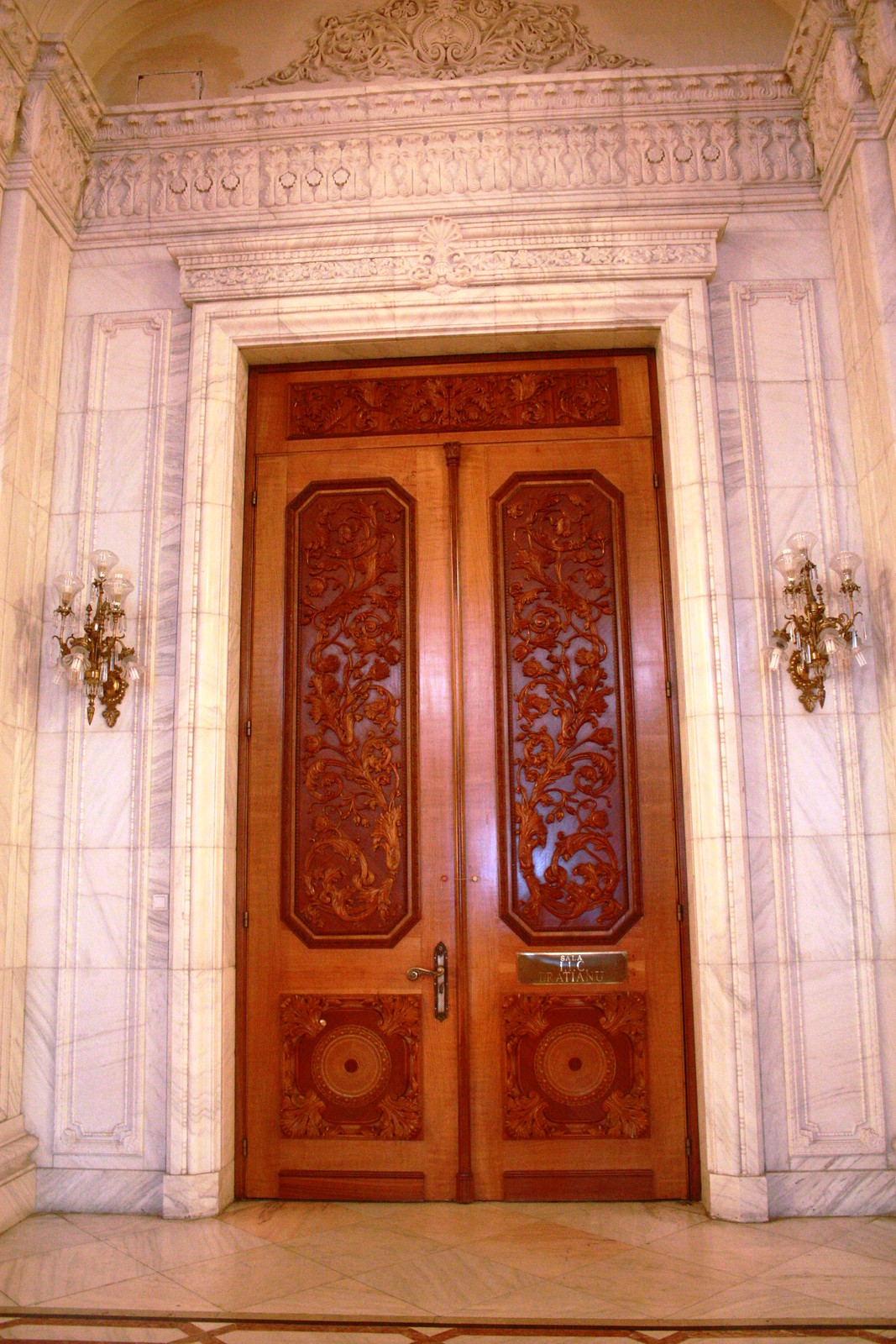The image showcases a grand entrance inside an opulent, possibly historic or governmental building, with elements reminiscent of a museum. The doorway, framed by white marble with intricate carvings at the top, features two imposing wooden doors approximately 20 to 30 feet high. Each door is ornately adorned with inlaid designs depicting branches, leaves, and figures carved in darker wood. The doors have symmetrical artistic patterns including circular ivy leaf motifs set within square panels at the bottom.

The left door has a handle, while the right door displays a small brass plaque that is difficult to decipher due to reflections. This area is additionally embellished with bronze etchings. Positioned about 60% up on the door frame are glass chandeliers, flanking each side and potentially illuminating the detailed work. The floor in front of the doors consists of brown tiles, adding to the grandeur of the setting.

On either side of the marble doorway, there are bronze lanterns that contribute to the ornamental and historic aesthetic of the entrance. The overall atmosphere suggested by the image is one of sophistication and rich architectural heritage, possibly indicating an entrance to a significant public building like a museum, castle, or government facility.